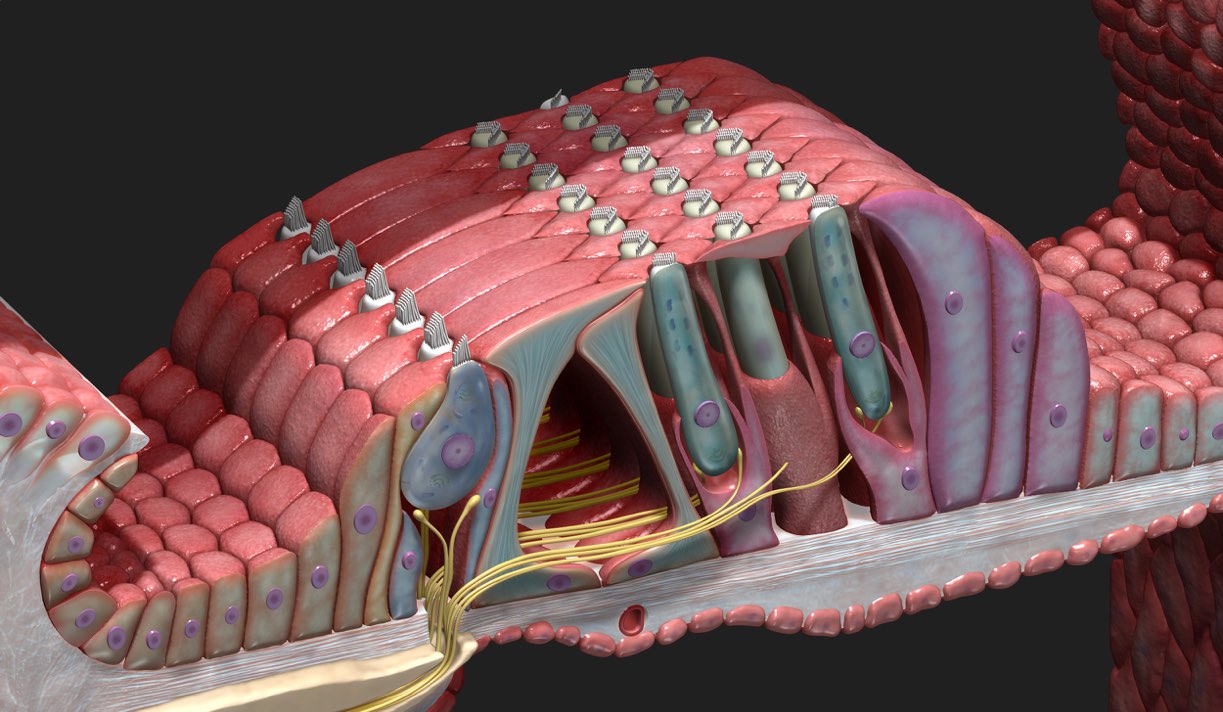This image is a close-up, three-dimensional rendering featuring a complex, layered structure against a black background. The prominent colors in the image are pink, gray, purple, and yellow. The object is positioned diagonally from the bottom left to the center right. The surface layer is primarily pink with multiple sectioned-off areas comprised of small, circular patterns that gradually increase in size and length from the top left to the bottom center.

Beneath these sections, the object's structure appears to be flipped over, revealing what lies underneath. It has a reddish-pink hue, reminiscent of scales, that separates into clearly defined sections. These sections have raised gray objects embedded in the pink material, arranged in four periodic rows across the surface. Each gray object surrounds a white bushing at its base, contributing to a textured, scale-like appearance.

On the side of the object, the structure appears aqua blue, rising in segmented sections adorned with similar dotted patterns. These features suggest a close-up view of an anatomical design or a biological model, possibly indicative of a muscle or connective tissue cross-section. Intriguingly, the central portion of the object includes a fibrous, yellow element that originates from the bottom left and extends horizontally along the bottom edge of the pink surface. The white cross-sectional areas beneath the pink surface reveal small purple dots and yellow tendrils connecting to the pink protrusions, adding to the intricate details of the rendering.